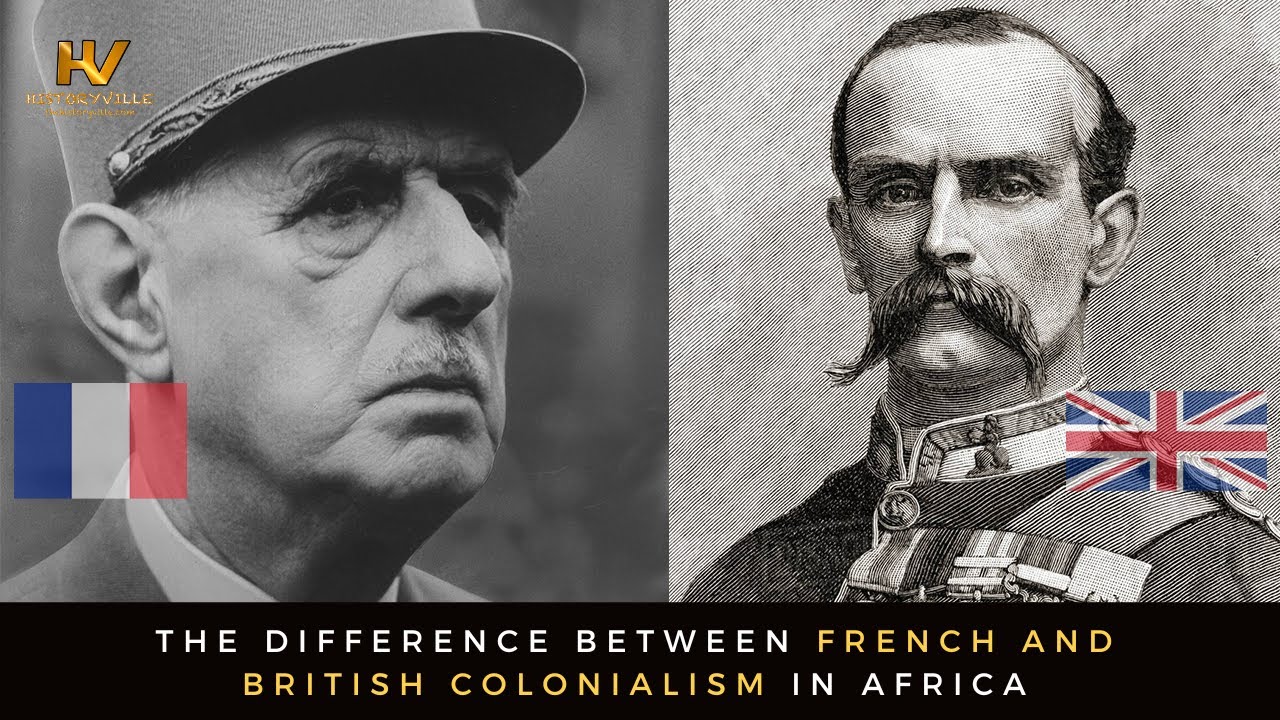This is an image pairing a black and white photograph with a pencil sketch, both depicting military or government officials. The left side features an elderly man in his 60s, captured in somber profile. He is distinguished by a military hat, prominent nose, small mustache, bushy eyebrows, and noticeable eye bags. A French flag is positioned next to his face, signifying his nationality. On the right side, a detailed pencil sketch portrays another official, likely from the 1800s to early 1900s, wearing a decorated military uniform adorned with medals. He is characterized by a pointed nose, thinning dark hair, and a full mustache that curves downward. The British flag is situated adjacent to his image. Below these visuals, set against a black background, is a caption in white text that reads: "The Difference Between French and British Colonialism in Africa."